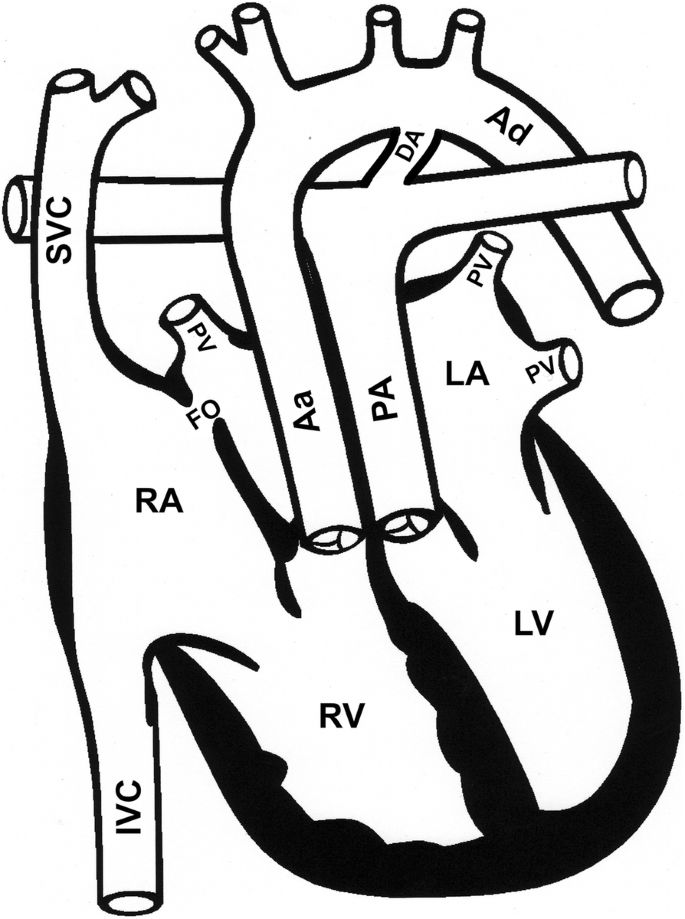The image is a black-and-white diagram of a human heart, professionally drawn with thick and thin lines on a solid white background. The heart's detailed structure includes two chambers at the bottom, labeled RV (right ventricle) and LV (left ventricle). Various tubes and vessels emerging from the heart are marked with acronyms such as IVC (inferior vena cava), SVC (superior vena cava), RA (right atrium), and LA (left atrium). Midway through the diagram, tubes labeled AA (ascending aorta) and PA (pulmonary artery) are depicted, with additional labels like FO, PV (pulmonary veins), DA, and AD scattered throughout. The overall illustration lacks shades of gray or color and is composed entirely of black lines on a white background.